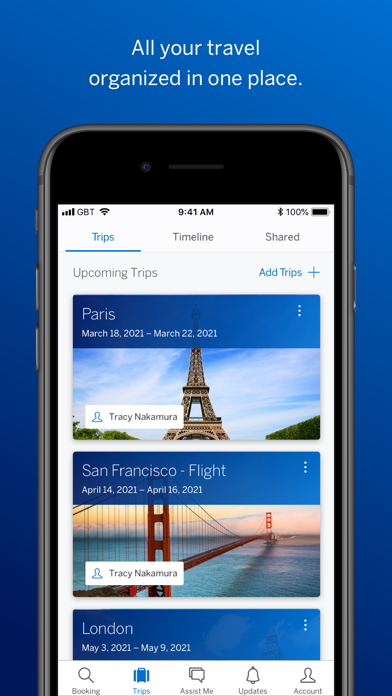A detailed caption for the image could be:

"In this vibrant illustration, a screenshot of an iPhone's travel organization app is shown against a blue background. At the top of the image, a bold header reads 'All your travel organized in one place.' Below this header, the iPhone display showcases three scheduled trips within the app. The first trip is to Paris, spanning from March 18th to March 22nd, 2021, and is accompanied by a small photo of the Eiffel Tower. Following this, a trip to San Francisco is listed from April 10th to April 16th, 2021, with an image of the iconic Golden Gate Bridge beneath it. The third trip is planned for London from May 3rd to May 9th, 2021; however, the screen cuts off before revealing its corresponding photo."